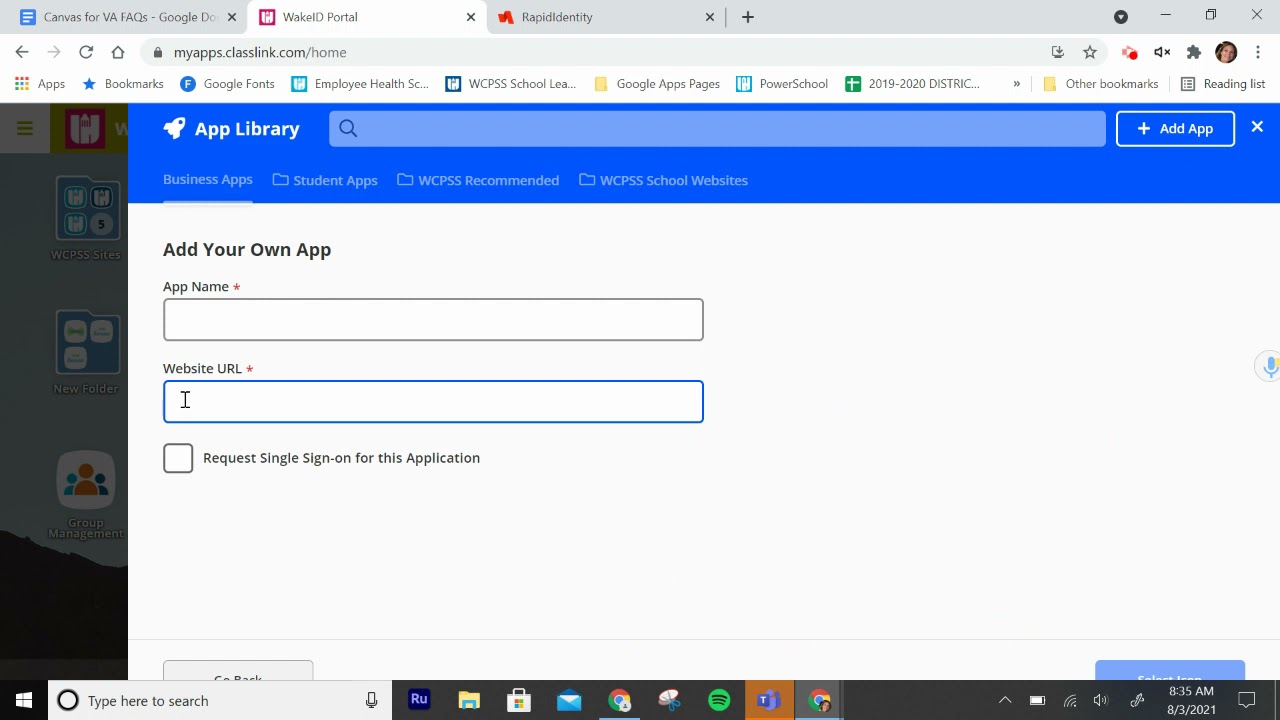The image appears to be a screenshot of a web dashboard from a website, possibly a portal for managing applications. 

**Top Section:**
- There is a light gray horizontal bar about an inch from the top.
- To the left, a blue square icon is followed by some text in black lettering.
- Adjacent to this, a white tab features a red square and more black text.
- Continuing right, a light blue section includes a tiny red icon and black lettering, ending with black 'X' and '+' signs.

**Search Bar Area:**
- Below the top section is a gray search bar displaying "myapps.classlink.com/home".
- On the right side of this bar, there are six clickable icons.

**Main Panel:**
- Directly beneath the search bar, a series of icons (ten in total) are aligned horizontally, each with a label.
- The left section of the dashboard has a blurred background where three app icons are vertically stacked on a light blue background fading to black at the bottom.

**Left Sidebar:**
- A blue-bordered area contains an outlined rocket icon labeled "App Library" at the top-left corner, followed by a long search bar.
- To the right of this, there is a section with a white border, blue fill, and a label "What App?" accompanied by a '+' sign to add an app and an 'X' to close.

**Add Your Own App:**
- In the left section, a partially faded white area features four dropdown options.
- Below this, a white area with bold black text states "Add Your Own App."
- There are fields for "App Name" and "Website URL," each accompanied by a large rectangle for input.
- Additionally, there is a white box with a black border containing the text "Request Single Sign-In for This Application."

**Bottom Bar:**
- The bottom border of the screen includes various icons.
- The date and time are displayed in the bottom-right corner.

This layout offers a comprehensive interface for adding and managing applications, complete with a search function, multiple clickable options, and a dedicated section for user-customized apps.